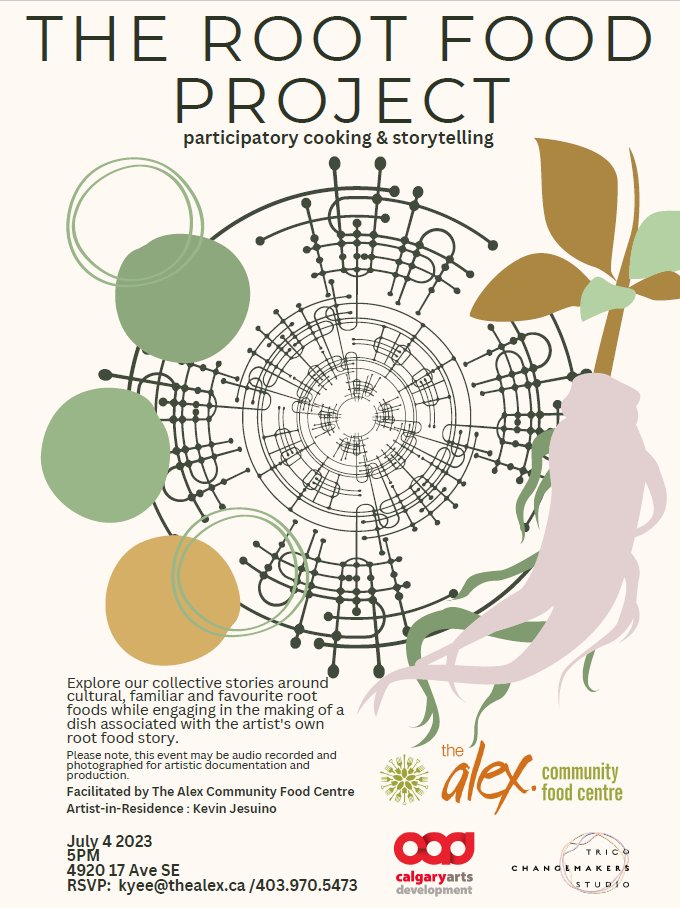The flyer for the Root Food Project features a vintage screen-printed design, dominated by a central circular motif with concentric circles and curving lines that resemble a cross between musical notes and a subway map with S-shaped paths and dots. Surrounding the central pattern are three solid circles - two sage green and one tan - interspersed with outlines of additional sage green circles. To the right, there is an abstract depiction of a pale purple ginseng root overlaying a sage green version, accompanied by a brown and sage green leaf. 

In large, bold letters at the top, the flyer announces "The Root Food Project" followed by "Participatory Cooking and Storytelling" in smaller text. Below the graphic, there is an invitation to engage in storytelling and cooking rooted in cultural and personal food traditions, with a note that the event will be recorded for artistic purposes. It provides the details: July 4th, 2023, 5pm, at 4920 17th Avenue SE. Interested participants are instructed to RSVP to KYEE at thealex.ca or call 403-970-5473. The event is facilitated by the Alex Community Food Center with Artist-in-Residence Kevin Jesuino. The lower portion of the flyer lists sponsors, including Calgary Arts Development and other unreadable names, reinforcing community involvement and support.